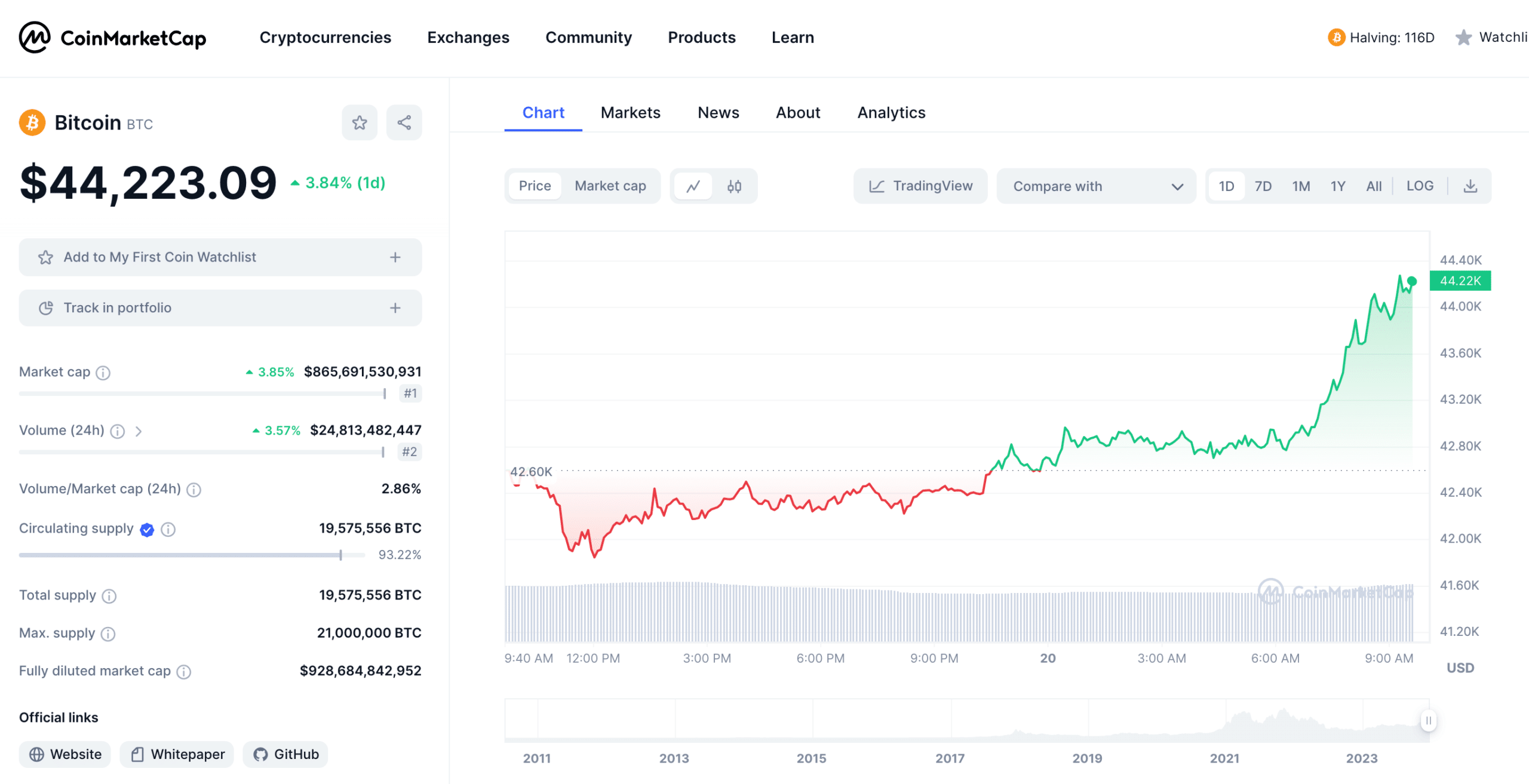The image depicts a trading website called Coin Market Cap. At the top left corner, the website's name and logo are prominently displayed, featuring a minimalist black 'M' next to the text "Coin Market Cap." Navigational tabs are situated at the top, including options such as "Cryptocurrencies," "Exchange," "Community," "Products," and "Lend." On the top right corner, the website displays a countdown labeled "Halving 116D" along with a "Watchlist" shortcut. 

The main content area showcases detailed information about Bitcoin (BTC). The current price of Bitcoin is highlighted in black, registering at $44,223.09. The percentage change, +3.84%, is prominently displayed in green. Users have the option to add Bitcoin to their watchlist via a button labeled "Add to My First Coin Watchlist," and track it in their portfolio.

Below the price data, key financial metrics are provided, including "Market Cap," "Volume / Market Cap," "24h Trading Volume," "Circulating Supply," "Total Supply," "Maximum Supply," and "Fully Diluted Market Cap." Off to the bottom left are official links to Bitcoin's website, whitepaper, and GitHub repository.

On the right side of the page, a detailed graphical representation of Bitcoin's performance is presented. The default view is a line chart, indicated by the blue color of the "Chart" tab, with alternative views available under tabs labeled "Market," "News," "About," and "Analytics." The line graph itself is color-coded, showing a red trend on the left half which transitions to a green, upward-trending line on the right half, indicating a recent positive trend in Bitcoin's market movement.